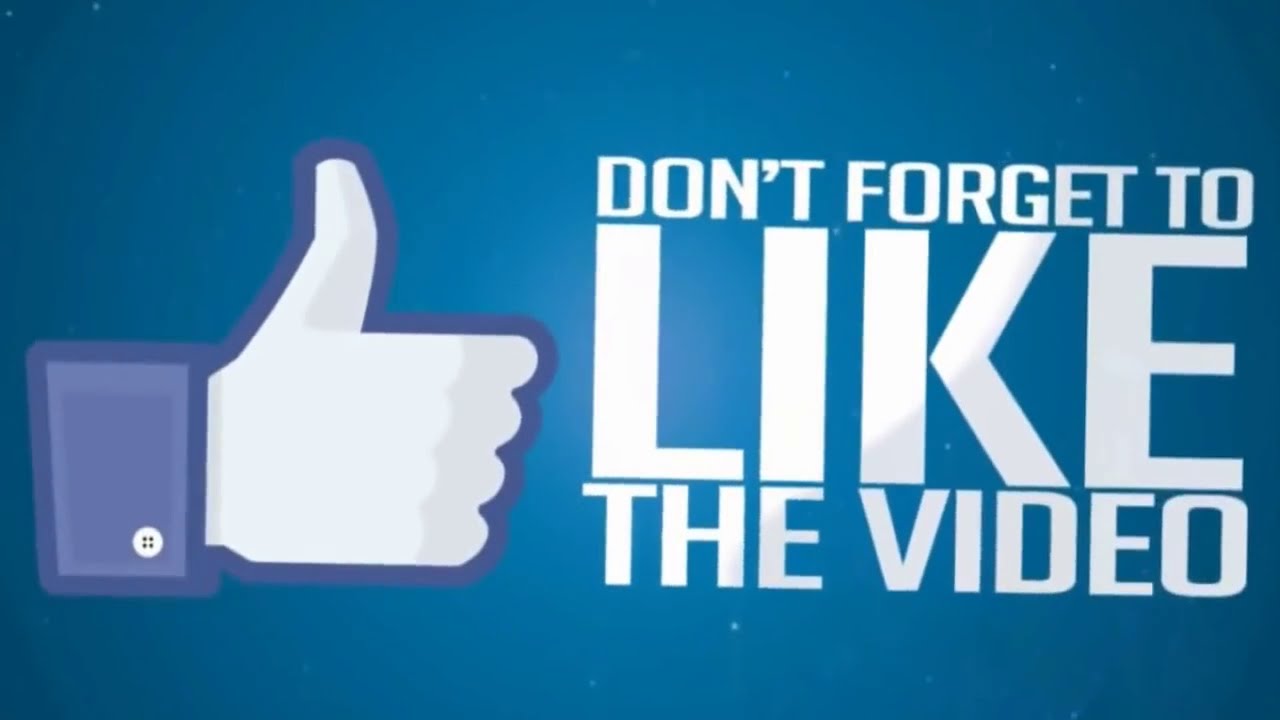The graphic image features a predominantly blue background with a subtle radial gradient, transitioning from dark blue at the edges to light blue at the center. On the left side of the image, there is a prominent thumbs-up icon reminiscent of the Facebook 'like' button. This icon, shaded in various hues of blue and white with gray accents, displays a white button on the shirt cuff at its base, adding a touch of realism. The thumb itself is outlined with a blue border, and there are shadowing effects on the knuckles and inside of the thumb. On the right side of the image, bold, white capitalized text says, "DON'T FORGET TO LIKE THE VIDEO," with the word "LIKE" significantly larger than the other words. The text has a slight transparency, allowing hints of the blue gradient background to show through. This composite image likely serves as a concluding screen for a video, encouraging viewers to engage and boost the content's visibility on social media platforms.